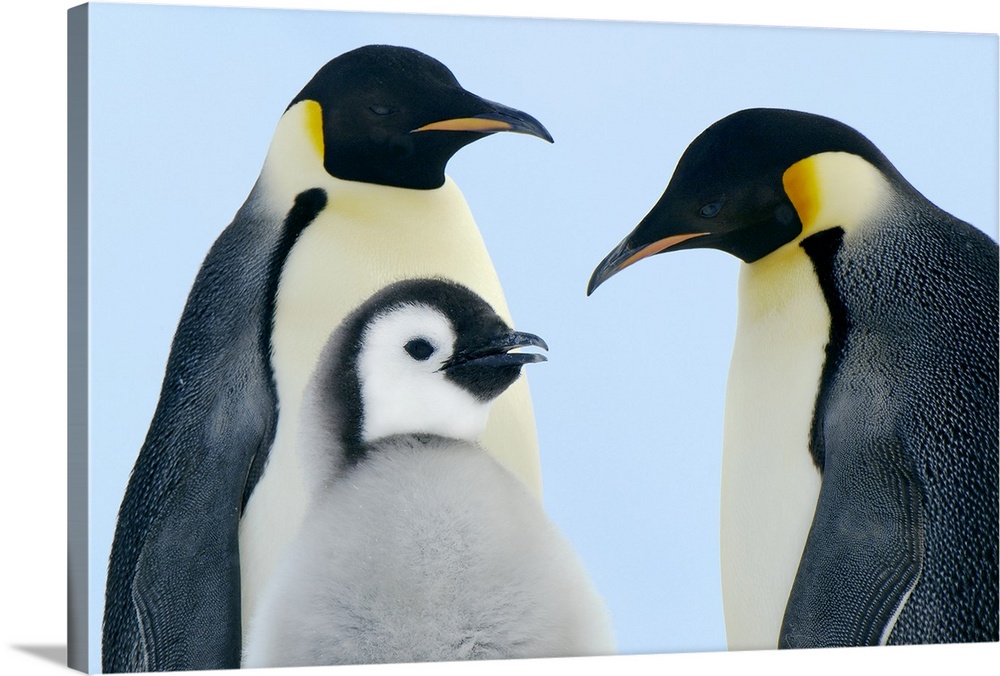In this image, set against a light blue background resembling the sky, three emperor penguins are prominently featured. Two adult penguins, characterized by their black heads, sharp black beaks with a bit of orange on the underside, and yellow streaks on the sides of their faces, are facing each other. Their bodies showcase a striking contrast, with white bellies, a transition of orange near their ears, and a grayish-black back with white spots. Between them, there's a fluffy baby penguin. This young penguin has mostly white fuzz around its face and body, dotted with a few black and gray feathers, especially on the top of its head. It also features a distinctive upside-down u-shaped black stripe arching over its head and extending to the back of its neck, and a stubby black beak. The adult penguins appear to be gazing at each other, while the baby looks towards the right side of the frame. The image exudes a touching scene of parental care within the framed artwork.